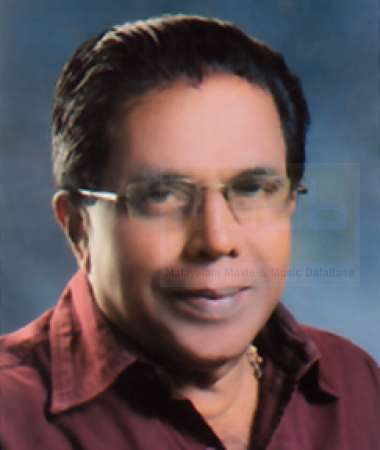This portrait photograph captures a middle-aged man of either Indian or Hispanic descent with light brown skin and black hair that is neatly combed back. He wears glasses and has a slight, closed-mouth smile. His shirt is a dark red, almost wine-colored, collared shirt, slightly open at the top revealing a gold chain around his neck. The background is a gradient of blue and gray, darker at the top left and fading to a lighter shade at the bottom right. The man is positioned from the top of his chest to his head and is staring directly at the camera with a slight rightward angle to his posture. The overall orientation of the image is a vertical rectangle, and the professional background gives the photograph a polished look.